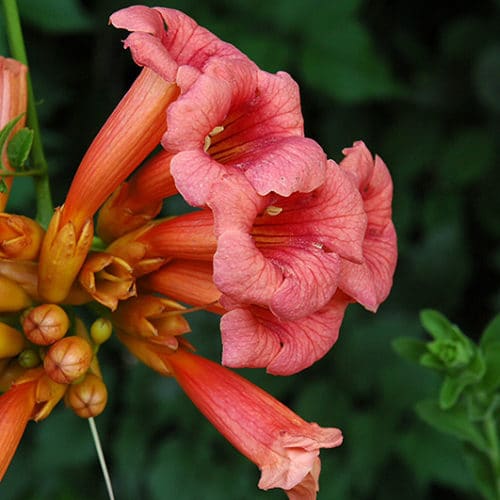This image features a cluster of striking coral-pink flowers, possibly resembling hibiscus but with a slimmer profile. A total of six flowers are in various stages of bloom, five fully opened with a sixth on the verge of blossoming. The flowers exhibit a range of pink hues from bright pink to salmon pink, and the lobes are distinct, each flower displaying five trumpet-shaped lobes that open and fold back, revealing circular centers. The flowers protrude gracefully from the left side of the frame, leaning slightly to the right. Each bloom is accented with a touch of yellow near its base. The background is a dense tapestry of dark green leaves, providing a vivid contrast to the colorful petals. This outdoor scene suggests a natural, lush setting, with the green foliage creating a verdant backdrop to the delicate pink and orange-red shades of the flowers.